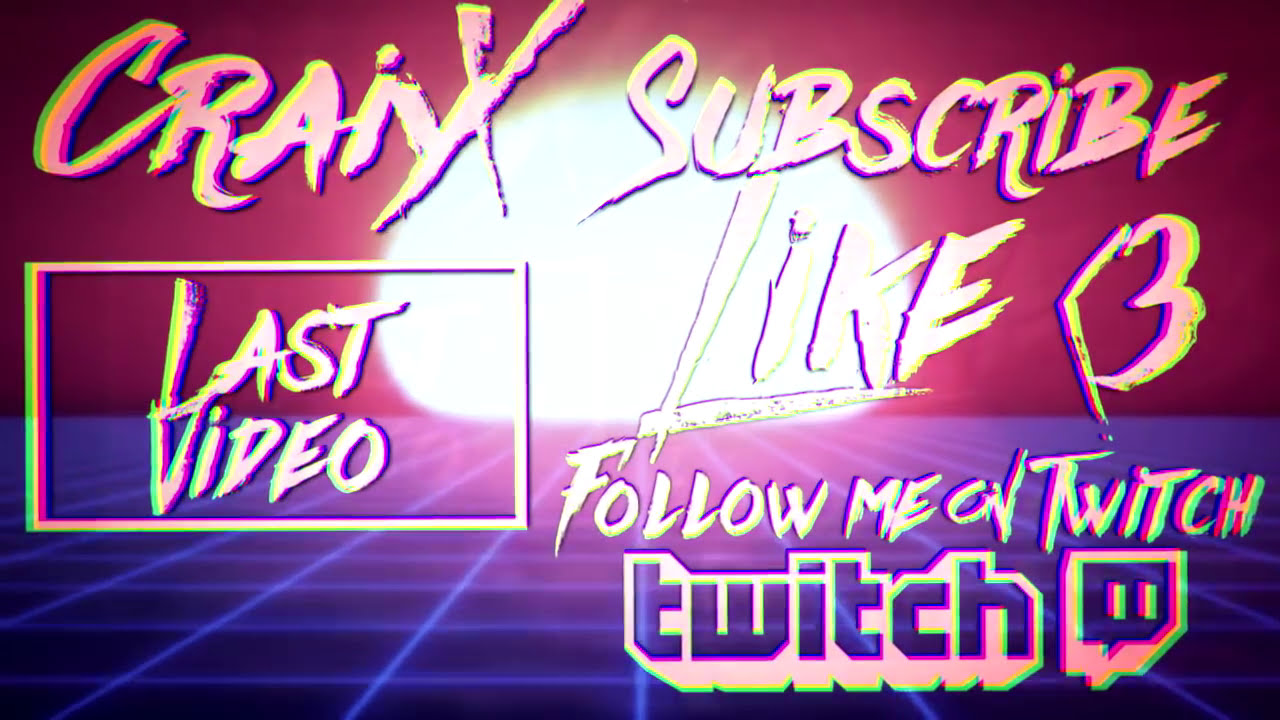This image captures a vibrant, cyberpunk-inspired advertisement, reminiscent of Disney's Tron. It features a neon blue, grid-like flooring that stretches towards a maroon horizon. At the juncture of the two, a large, glowing, slightly oval sun dominates the center. Boldly colored, the background transitions from deep blue grids to a purpley fuchsia sky. 

In the foreground, several text elements are scribbled prominently. The top-left reads "CRANX" or possibly "CRAI-X" in all caps. To the immediate right is the word "SUBSCRIBE" in large, uppercase letters. Below "CRANX" is a small box containing the text "LAST VIDEO." Below "SUBSCRIBE," a sequence reads "LIKE > 3 FOLLOW ME on Twitch," accompanied by the Twitch logo. This setup resembles the end screen often found on YouTube videos, prompting further interaction.